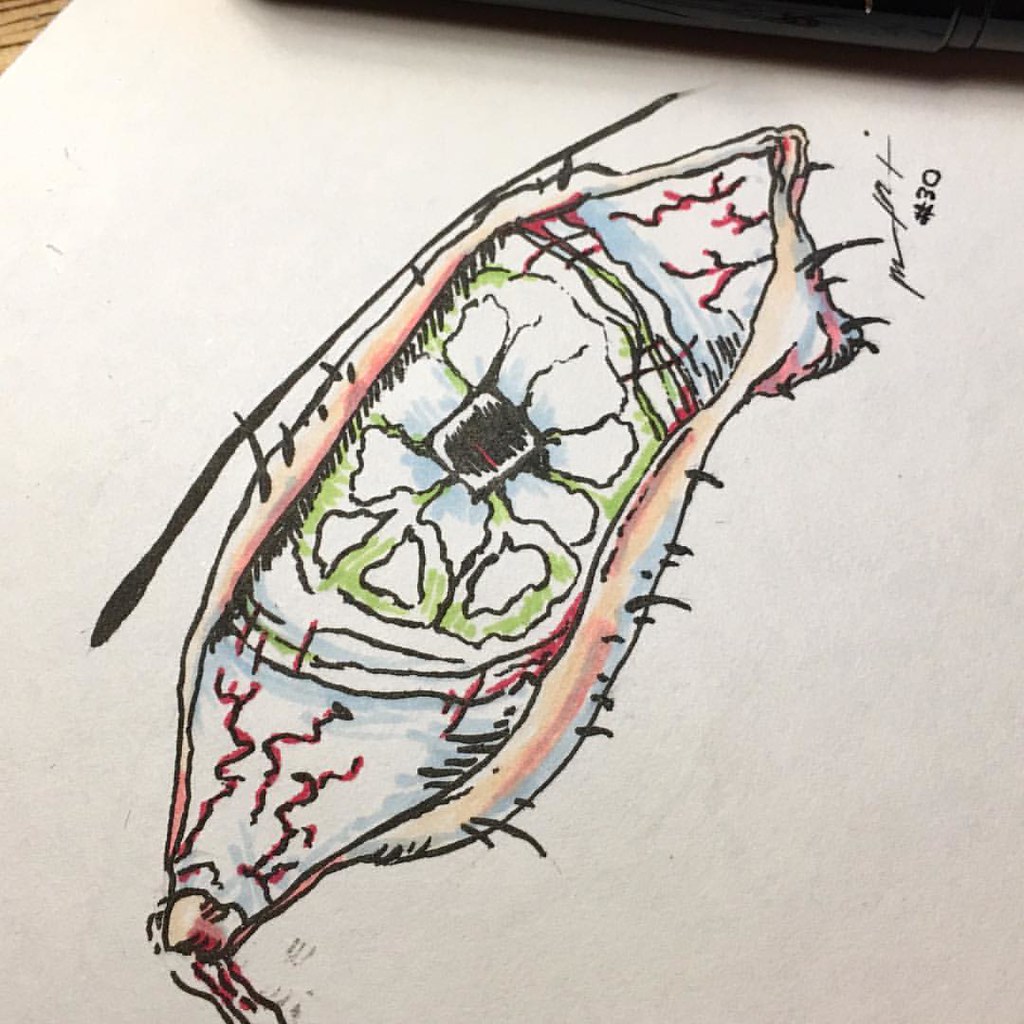This is a detailed and vivid square photograph of a drawing rendered in markers on a white, thick piece of paper. The drawing, slightly tilted to the left, features an eye as its primary subject. Located in the upper right-hand corner is a neat signature in black ink. The eye's design deviates from a typical representation; the sclera is bloodshot, especially at the corners, enhancing a sense of intensity or fatigue.

In an imaginative twist, the iris of the eye adopts a floral pattern with a backdrop of green, giving the illustration an otherworldly feel. The eyelid is meticulously shaded with a gradient of light and dark flesh tones, contributing to the realistic depth and dimension of the piece. Scattered sporadically throughout the drawing are patches of light blue and dark pink, adding abstract elements to the composition.

The main structure of the eye is outlined and detailed in black marker or pen, emphasizing the stark contrasts and defining features. The eye itself is oriented so that the inner corner is situated at the lower left-hand side of the image, while the outer corner extends towards the top right quadrant. The entire artwork, with its rich colors and intricate details, is set against the thick white paper background, providing a striking contrast that highlights the drawing's uniqueness and creativity.